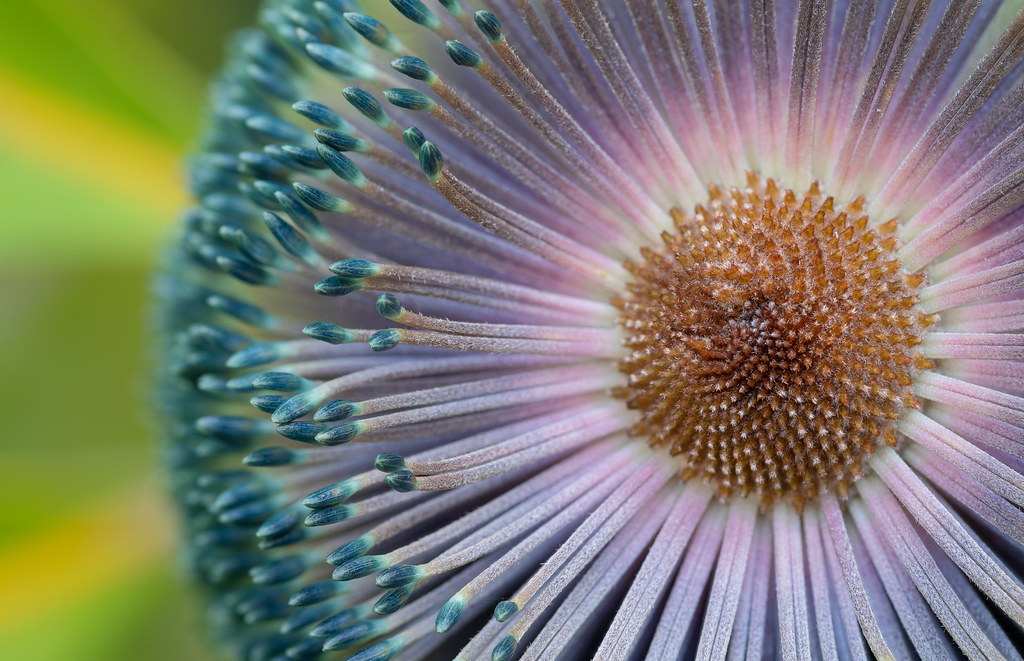This close-up photograph showcases the intricate details of a flower's center. The core of the flower, a circular area filled with amber and brown pollen, serves as the focal point. Radiating from this central point are numerous filaments or stems, possibly over a hundred. These structures display a gradient of colors: starting as white at the base, transitioning through shades of pink, lavender, and purple, and culminating in tips that range from bluish to teal, sometimes with green buds at the very ends. The stems have a notably grainy texture, resembling tiny matchsticks. The background is artfully blurred, consisting of various shades of green and soft yellow hues, enhancing the flower's vivid details and suggesting an outdoor setting. The overall composition gives the flower a dynamic, almost otherworldly appearance, with a pattern reminiscent of cilia or spores.